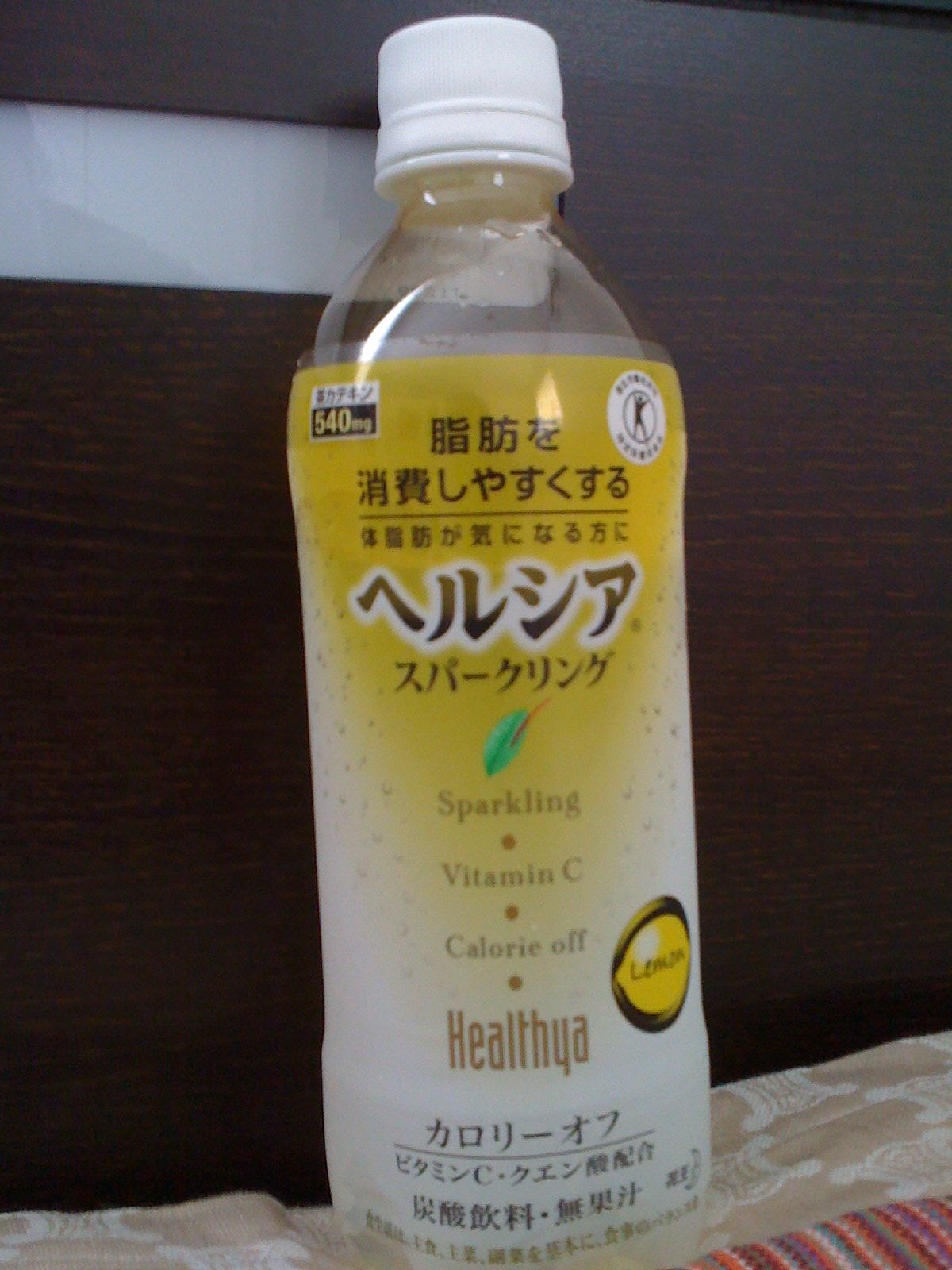The image features a clear plastic bottle containing a lemon-flavored sparkling juice, centered prominently. The bottle has a white cap and a label that transitions from yellow at the top to white at the bottom. The label displays various text, including some Asian characters, with English words like "sparkling," "vitamin C," "calorie off," and "healthier." To the right side of the label, there's a black circle with a yellow lemon image and the word "lemon" written in black text. 

The background showcases a dark black wooden panel adorned with lighter brown wood grain patterns, possibly indicating it's part of a wall, such as a headboard. There's a rectangular white cutout extending from the center of the image to the left, which appears to be frosted glass or plastic. The bottle rests on a peachy tan fabric with white shapes, potentially bedding, and the bottom right corner of the image displays a colorful piece of additional fabric or material, adding a vibrant touch to the composition.